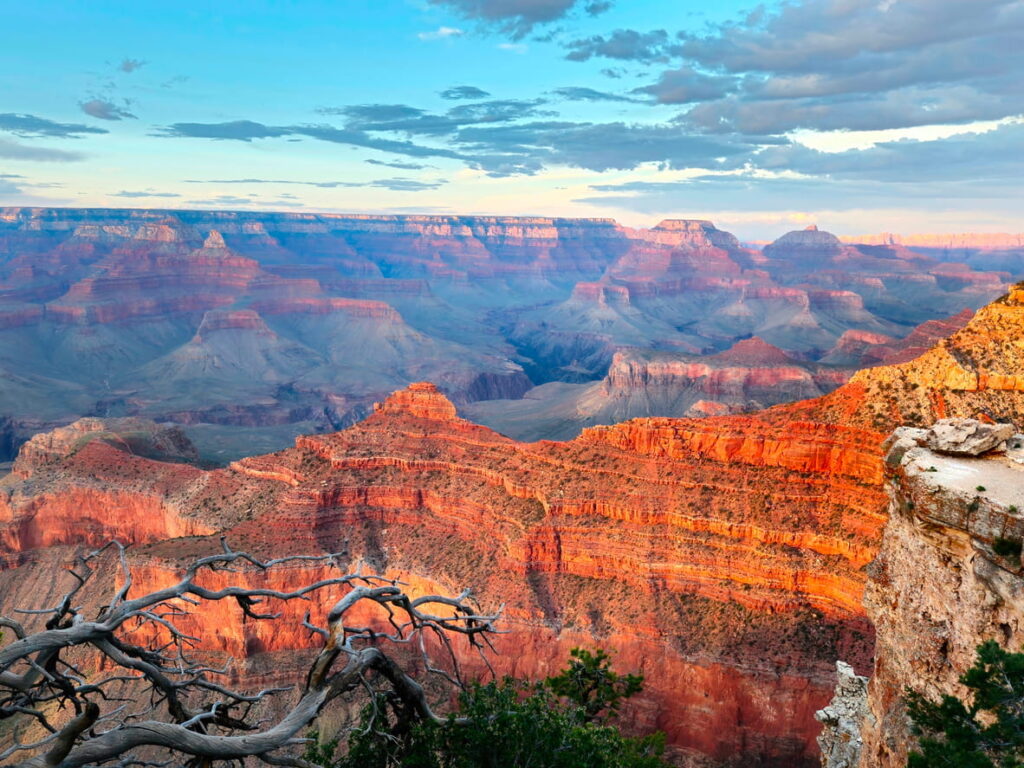The image captures a stunning, vibrant aerial view of a canyon area, possibly resembling the Grand Canyon or other mountainous terrain in the western United States. The picture highlights an array of striking colors including shades of orange, red, beige, gray, and brown, with the canyons displaying layered rock formations bathed in natural sunlight. The foreground reveals tree branches and green leaves, adding a touch of greenery to the rugged landscape. The sky in the background is partly cloudy, with most clouds concentrated towards the right side of the image. The scene is vividly clear, showcasing the bright, natural light and the intricate details of the canyon’s rocky structures. There are no texts or numbers on the image, enhancing its pure depiction of natural beauty.